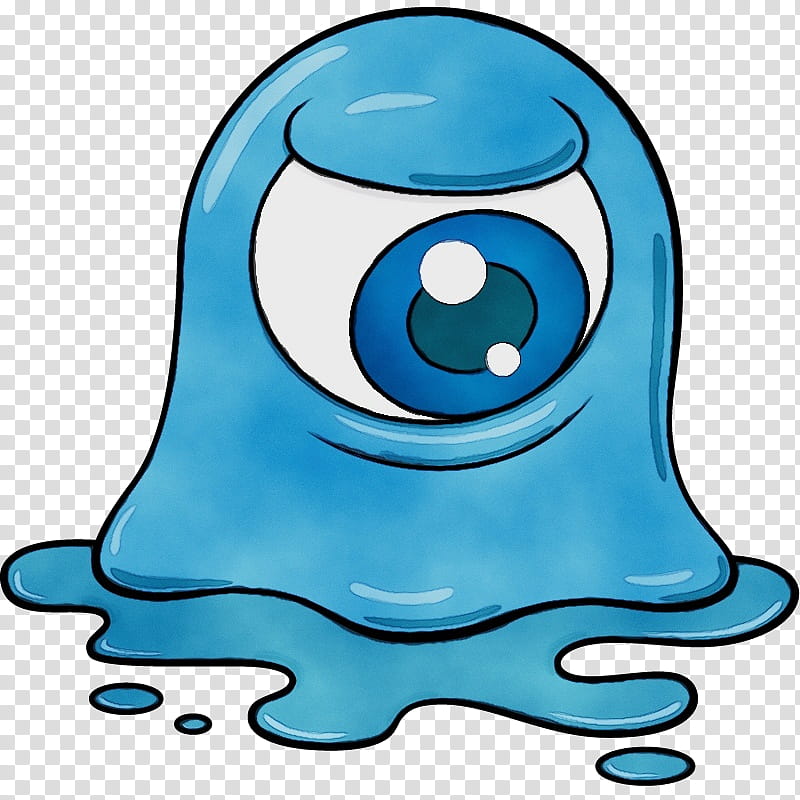This illustration depicts a light blue, gelatinous blob resembling a ghost with a single, large eye, centrally located and prominently featured. The character's body shape is both short and wide, with a melting, flowing form extending into a puddle beneath it, accompanied by several small drops of the same light blue hue. The eye itself, enormous and almost half the size of the blob, has a light blue pupil with a darker blue-green center, highlighted by white areas that enhance its cartoonish and expressive appearance. The shading on the blob, with light blue and darker blue teal tones, gives it a three-dimensional and shadowed effect. The background consists of a checkered white and gray pattern, indicating a transparency suitable for easy editing. This whimsical and slightly melancholy figure evokes a likeness to the ghostly slimes seen in the Ghostbusters movie.